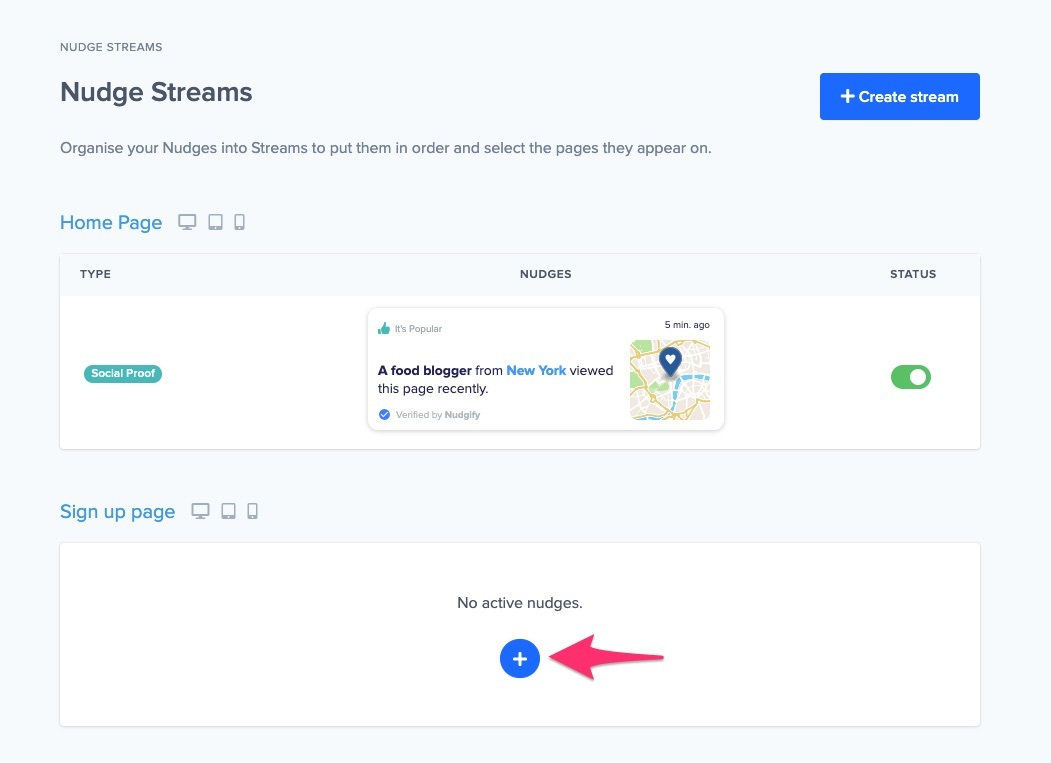The image depicts a user interface layout for organizing nudges. 

In the upper left corner, the phrase "nudge streams" is displayed twice, once in a smaller font and once in a larger font. On the same level but to the right, there is a blue button labeled "Create Stream" accompanied by a plus symbol. 

Below, there's instructional text explaining that users can "organize your nudges into streams to put them in order and select the pages they appear on." The word "homepage" is highlighted in teal, indicating its active status. Images of a computer monitor, a tablet, and a phone illustrate the application across various devices.

Further down, a section labeled "Type" displays "Social Proof," and in the "Nudges" section, there is a message stating "This is popular" accompanied by a green thumbs-up icon. It informs that "A food blogger from New York viewed this page recently," which is verified by Nudgify, marked by a blue circle with a white check mark. A small map with a heart icon shows the location, noting the action occurred five minutes ago.

On the right side, under "Status," there is a green toggle indicating that the feature is active. Below that, in the "Signup Page," icons for a computer monitor, tablet, and cell phone are shown again. The field states "No active nudges," marked by a circle with a plus sign, and a red arrow points to this area, suggesting it as a focal point for user action.

It appears this interface is designed to educate users on how to manage and organize their nudges effectively.